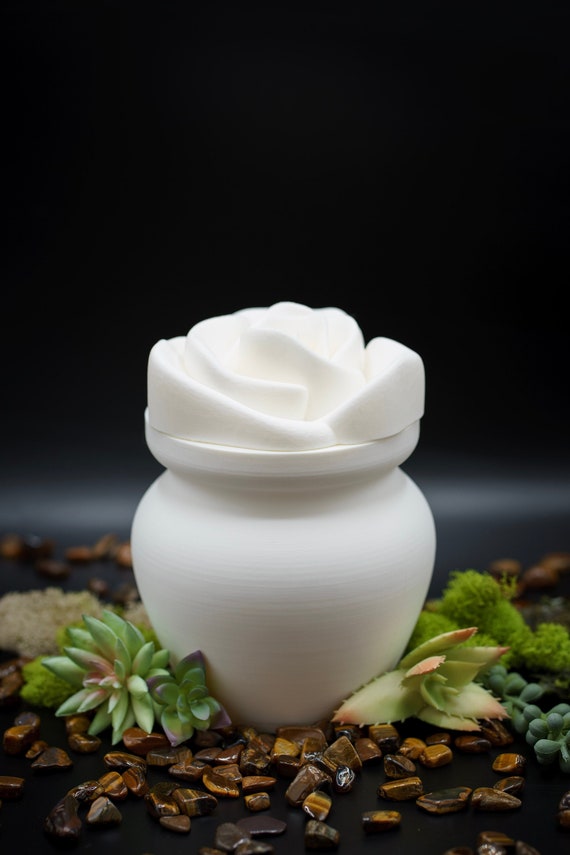In this photograph, a white ceramic planter sits elegantly on a bed of shiny pebbles in various shades of brown—ranging from light to dark, some even striped. The planter is topped with an intricately designed lid resembling a blossoming flower which appears almost like white petals, lending it a decorative flair. Surrounding the base of the planter are lush green succulents; on the right side, light green plants with sharp spikes, and on the left, a combination of darker green leaves, with hints of pink and gray. The background of the image is predominantly black, transitioning to a thin gradient of light and dark gray towards the middle and bottom, enhancing the planter’s prominent display. The scene is arranged on a sleek, black surface, amplifying the overall sophistication of the display.